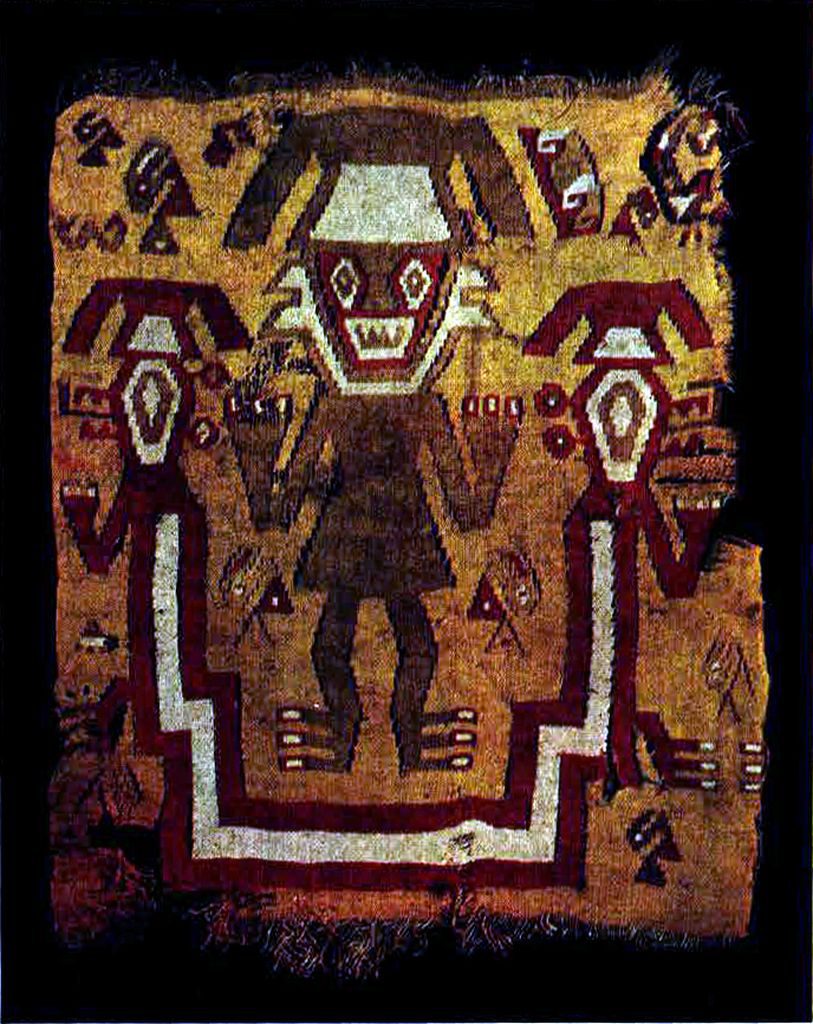This photograph showcases a detailed and vibrant piece of textile art, likely a part of South or Central American indigenous cultural heritage, possibly Peruvian or related to Aztec culture. The main focus of the textile is a central humanoid figure, distinguished by its striking features. It has three fingers on each hand and three toes on each foot, with the toes extending laterally and the hands raised above the head, resembling claws with white nails. The figure sports a headdress or mask featuring angular, diamond-shaped eyes with black pupils and white surrounding areas, and a mouth showing three sharp, white teeth.

Surrounding the central figure are intricate geometric designs and symbols, predominantly using a palette of browns, whites, and a touch of red against an orange-brown background. A white sash or strip with diamond patterns extends downward and arcs around the figure. Despite its age, with parts of the material frayed and pieces missing, the textile's craftsmanship remains evident, including detailed embroidery and fringes along the top and bottom. The work of art rests against a black backdrop, which enhances the richness and depth of its colors and designs.